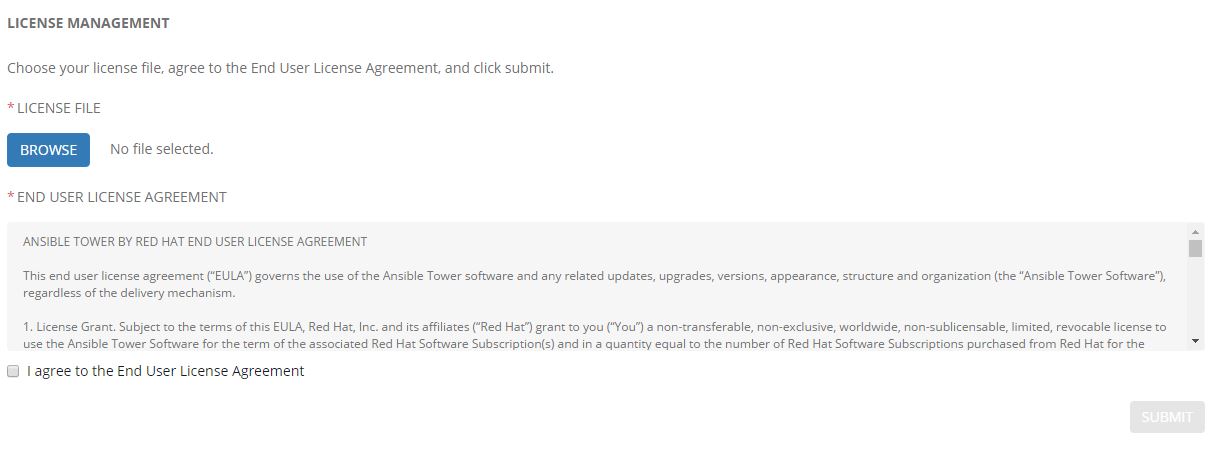### Detailed Caption:

The image depicts a webpage interface under the category of "Websites," specifically for "License Management" within an Ansible Tower by Red Hat environment. The webpage is predominantly white, set against a blue background. At the top, bold text reads "License Management," followed by the instructional text: "Choose your license file. Agree to the end user license agreement and click Submit."

Below this, there is a section labeled "License File," accompanied by a button labeled "Browse." The "Browse" button is blue with white lettering, indicating interactivity. Adjacent to it, there is text stating "No file selected," suggesting that no license file has been chosen yet.

Beneath these form elements, there is a gray square that contains the text "Ansible Tower by Red Hat End User License Agreement." The agreement details the governing terms for the use of the Ansible Tower software and covers various aspects such as updates, upgrades, versions, appearance, structure, or the organization of the software, delivered by any mechanism.

The first section of the license agreement is titled "License." It states: "Grant subject to the terms of the EULA, Red Hat, Inc., and all its affiliates." It further explains that Red Hat grants the user a non-transferable, non-exclusive, worldwide, non-sub-licensable, limited, revocable license to use the Ansible Tower software. This license is valid for the duration of the associated Red Hat software subscriptions and is limited to the quantity equal to the number of Red Hat software subscriptions purchased from Red Hat.

This webpage appears to be part of the user interface for managing software licenses, ensuring compliance with the terms set forth by Red Hat, and facilitating the upload of license files necessary for the operation of Ansible Tower.